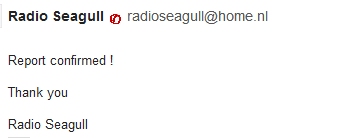This image features a message on an all-white background, seamlessly blending in with the rest of the page. At the very top, there is a bold black text stating "Radio Seagull," accompanied by a small red logo—a circle with a line through it. To its right, in a smaller, non-bold font, the text reads "Radio Seagull at home dot nl." Concealed to the left and faintly visible, there's a vertical blue line. Below this heading, the text "Report confirmed!" is displayed, followed by "Thank you." Finally, the message concludes with the text "Radio Seagull," all presented in the same regular font style. Another faint blue line runs horizontally beneath this last "Radio Seagull."